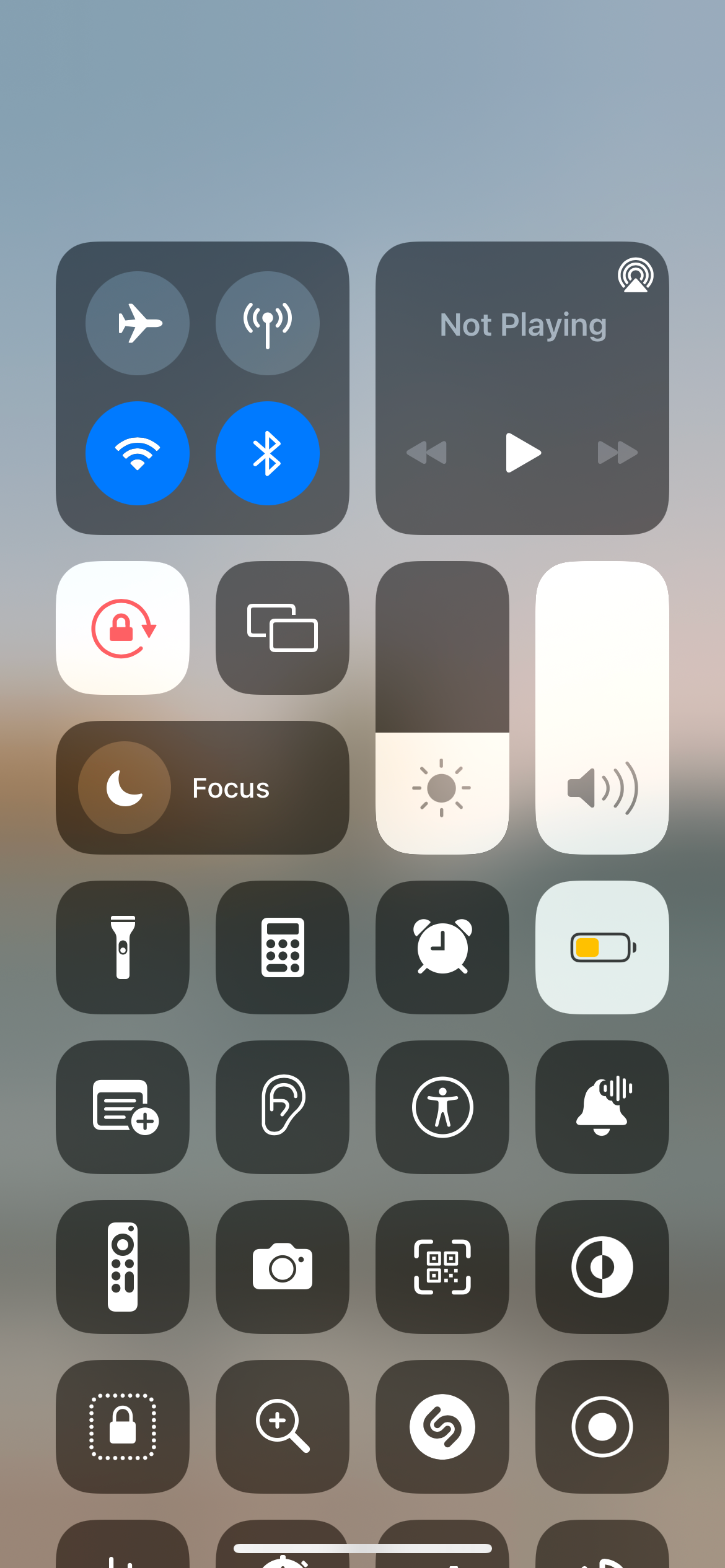In this image, captured from an Apple iPhone, the screen displays the Control Center interface. The Control Center is overlaid on a blurred background that is predominantly blue, although the exact details of the background image are indistinct. 

The Control Center is divided into various sections, each containing different icons and shortcuts. The top of the Control Center features a section related to connectivity. This section includes several icons: an airplane symbol indicating Airplane Mode, a cellular data icon, a WiFi symbol, and a Bluetooth symbol. Both the WiFi and Bluetooth icons are highlighted with blue circular backgrounds and white symbols, suggesting they are active.

Below the connectivity icons is a media control box displaying the message "Not Playing" in grey text, indicating that no media is currently being played.

Further down, other functional shortcuts are visible. These include:
- A screen rotation lock icon
- A screen mirroring icon
- A focus mode icon
- A brightness adjustment slider
- A volume control slider

Additional icons for utility functions include shortcuts to the calculator, clock, and a few other applications or tools that are not explicitly identified in your description but are present in the Control Center.

Overall, this detailed screenshot provides a glimpse into the various quick-access functions available on an iPhone's Control Center, showcased against a softly blurred blue background.